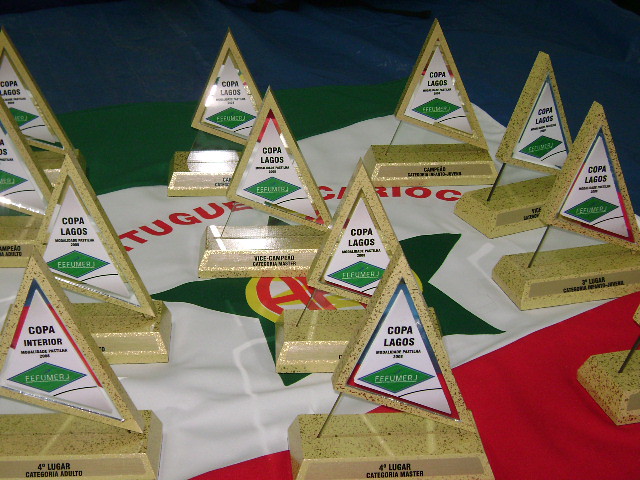The color photograph captures a collection of twelve trophies arranged meticulously in three rows of four on a table adorned with a striking flag. The trophies, primarily for the Copa Lagos beach soccer tournament, have an elegant design featuring a triangular, sail-like top supported by a thin rod anchored into a stone-like base that resembles a gold brick. These bases contain plaques with inscriptions like "4th Lugar Categoria Master," indicating various placements in the competition. The tablecloth underneath sports a flag design with a green stripe at the top, a thicker white stripe in the middle, and a red stripe at the bottom, complete with a green star centered in the white area. The intricate design of the trophies, coupled with the vivid colors of the flag and the detailed inscriptions, makes the scene both visually striking and significant.